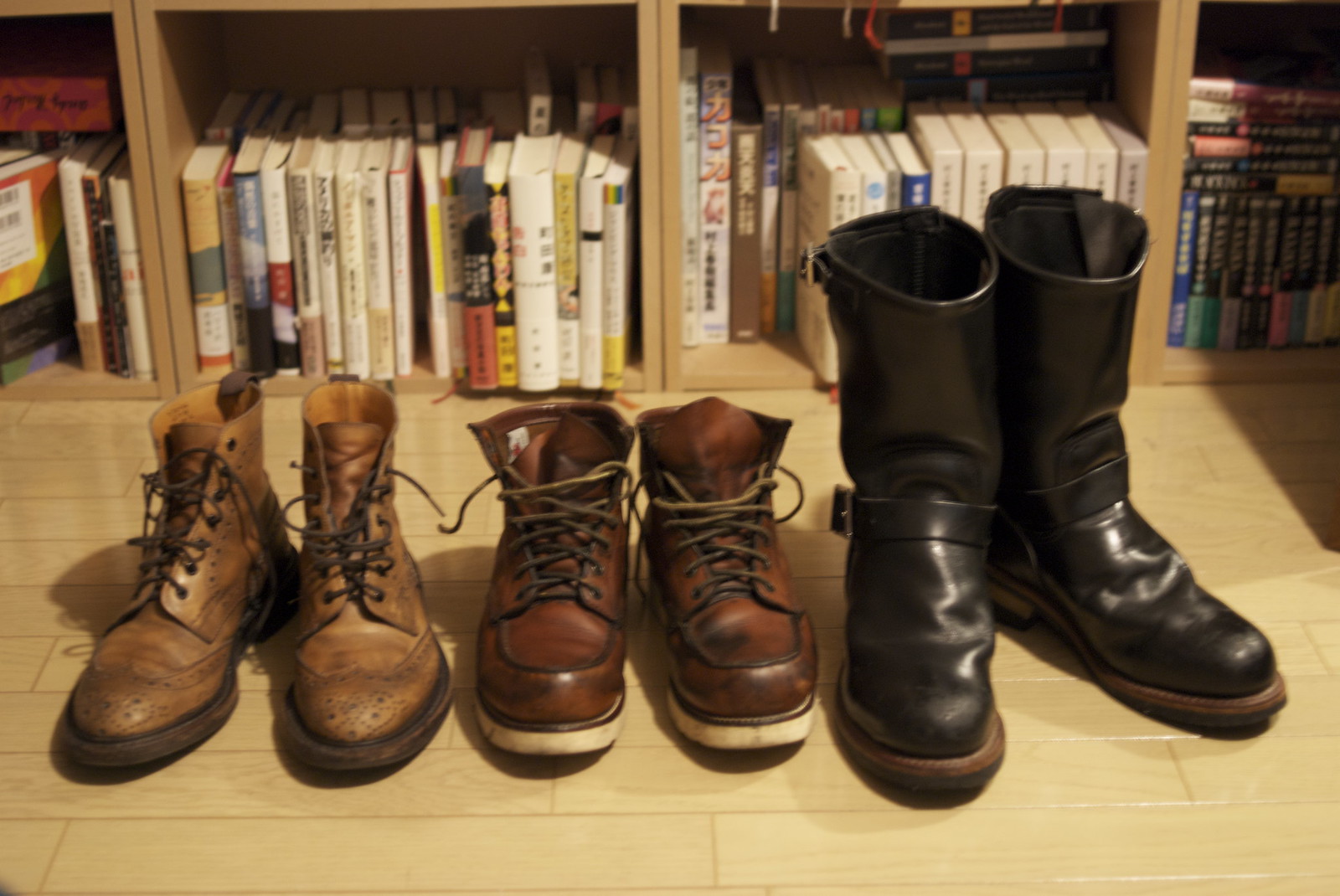The image showcases a light blonde wood plank floor set horizontally, supporting three distinct pairs of boots. Nearest to the foreground is a tall, buckskin-colored dress boot with wingtip tops and cord ties extending up to the calves. Beside it stands a pair of sturdy, dark brown work boots with yellow cord ties and a white-colored sole, reaching ankle height. The third pair is a tall, black motorcycle boot featuring a strap and buckle across the ankle, rising to the calves. In the background, a bookshelf made of the same light wood as the flooring is densely packed with books of various sizes and colors, including notable hues of white, red, and blue.